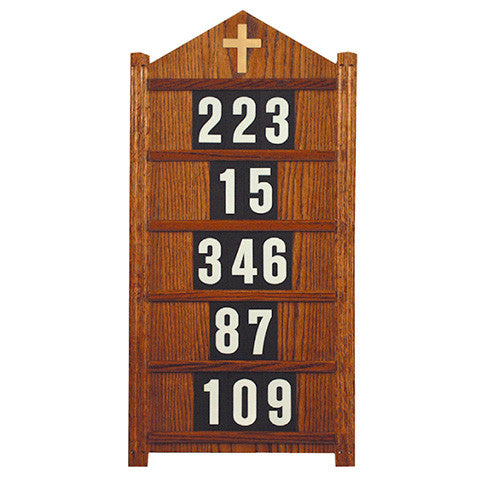This image depicts an old-fashioned wooden church placard, rectangular and vertically oriented, featuring a pointed triangular top crowned with a brass-looking cross. The placard is divided into six sections by two vertical bars, with the numbers 223, 15, 346, 87, and 109 displayed in white on a black background. These numbers are housed in compartments supported by horizontal bars, suggesting they can be changed out. While primarily believed to have been used to track weekly attendance, it's possible the board also recorded information such as tithing amounts or sermon statistics. The placard's traditional design, including trim on both sides and its prominent cross, hints at its longstanding place within church history and Christian symbolism.